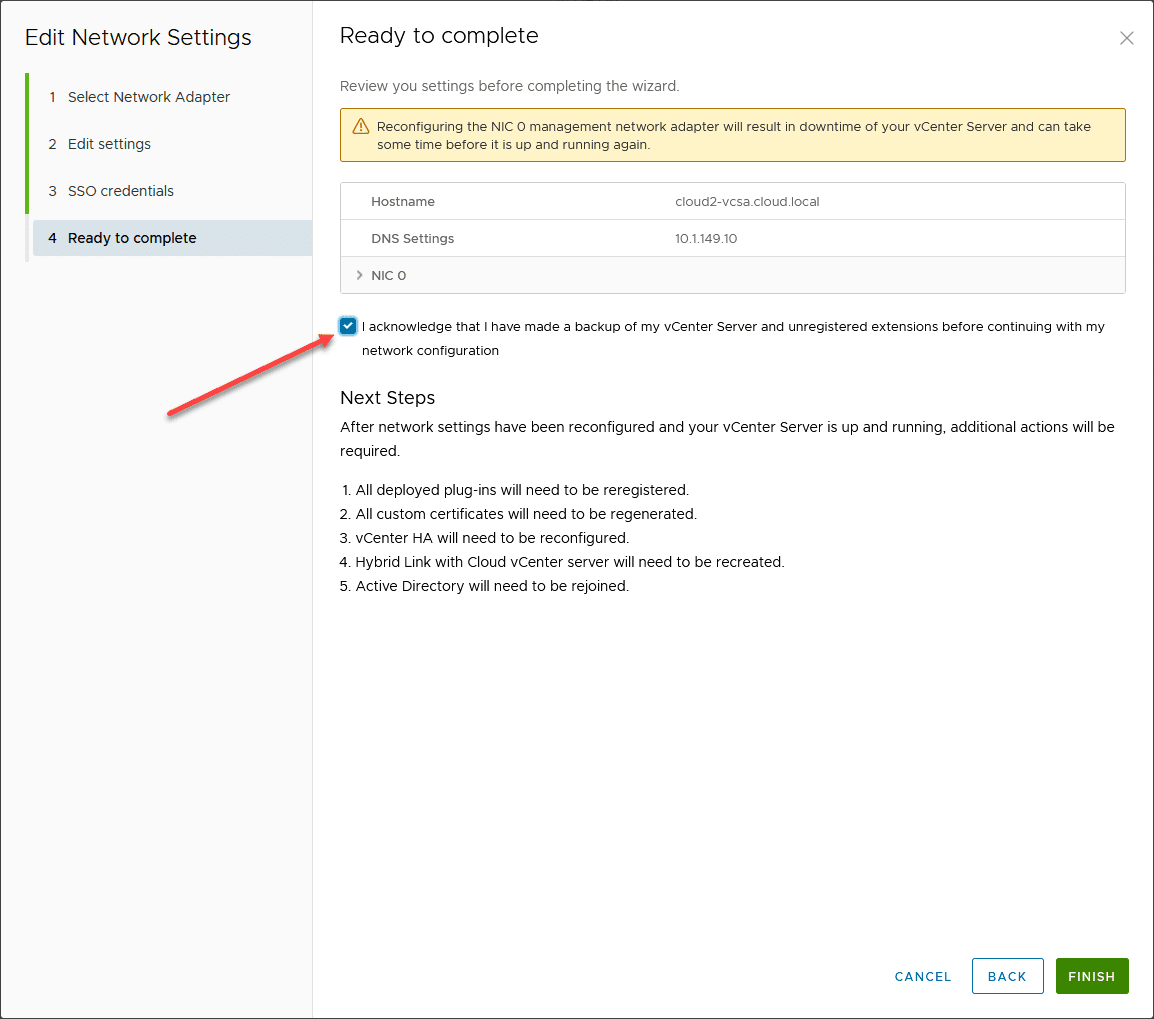This image depicts an open software window with a white background, entitled "Edit Network Settings." The window breaks down the process into four sequential steps: "Select Network Adapter," "Edit Settings," "SSO Credentials," and "Ready to Complete," displaying the progression on a column to the left. Currently, the highlighted step is the fourth one, "Ready to Complete."

Adjacent to the progression column, a confirmation message reads: "I acknowledge that I have made a backup of my vCenter server and unregistered extensions before continuing with my network configuration." Next to this message, a blue checkmark is prominently displayed with a red arrow pointing towards it, emphasizing the importance of the acknowledgment.

In the bottom right corner, the user interface offers three action buttons: "Cancel" to exit without saving changes, "Back" to return to the previous step, and "Finish" to complete the process. The overall layout suggests the user is finalizing network configuration settings, specifically for a vCenter server environment.